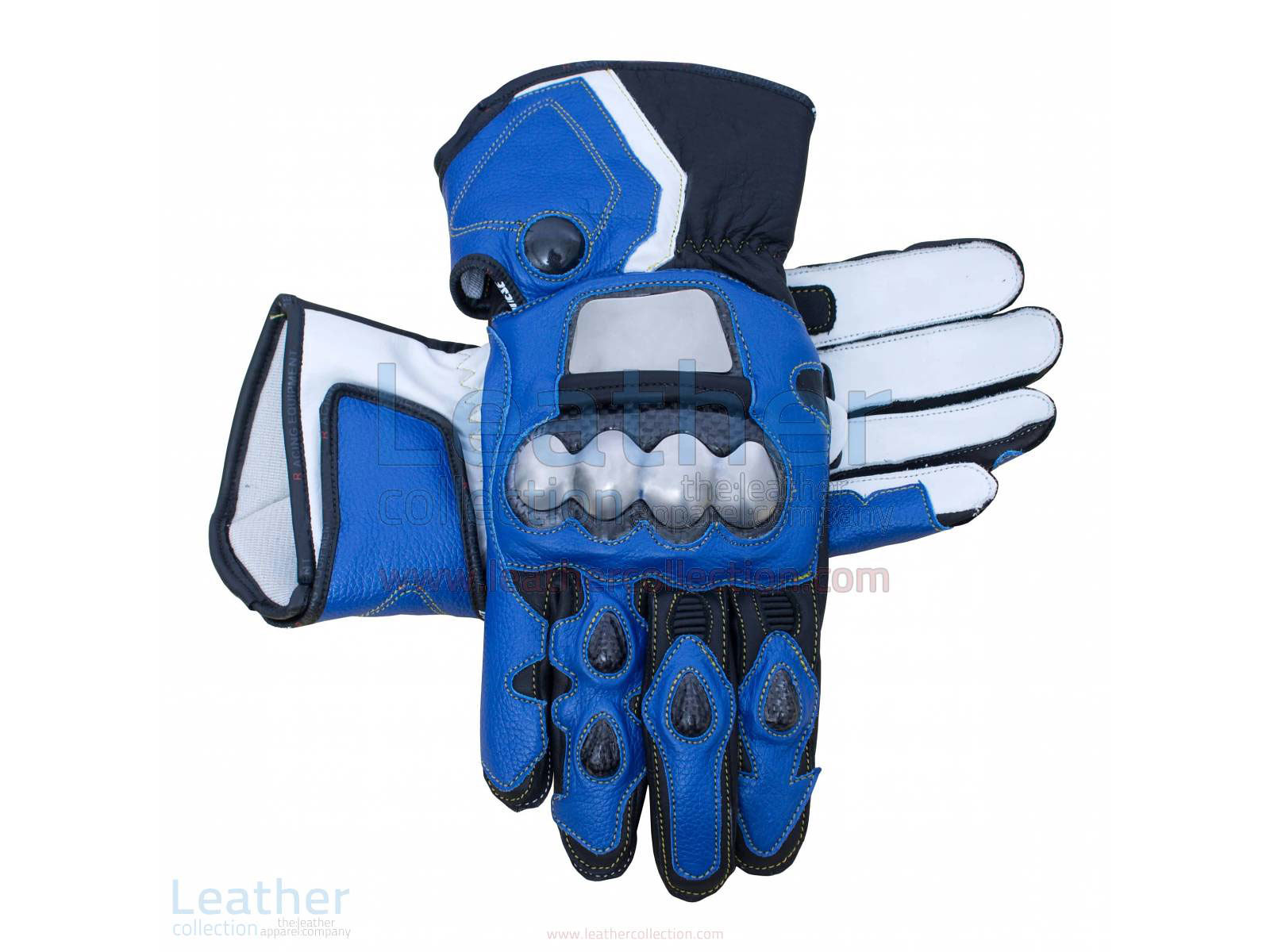This image features a pair of royal blue leather gloves with distinctive black trim and white detailing. The left-hand glove lies on the bottom with its palm facing up, revealing a completely white palm area with blue trim along its edges. The right-hand glove lies on top with its palm facing downwards, displaying intricate white markings mimicking knuckles and black trim around the cuffs. Both gloves are heavily padded, indicating they are suitable for activities like skiing or biking. The background of the image is entirely white. In the bottom left corner, blue lettering spells out "Leather Collection," while centered at the bottom in black is the URL "www.leathercollection.com." The gloves prominently feature round, knob-like black buttons at the wrist.